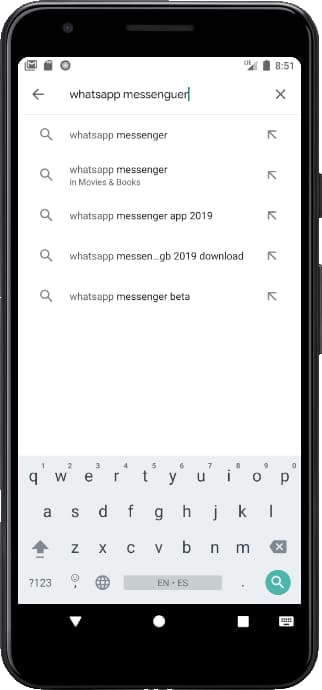In the image, we observe a smartphone screen displaying the search interface of an app store, likely the Google Play Store. The main focus is on the search results for "WhatsApp Messenger." The screen shows a list of search suggestions including "WhatsApp Messenger app 2019," "WhatsApp Messenger GB 2019 download," and "WhatsApp Messenger beta." 

At the top of the screen, the phone's status bar reveals an "A51" device, a battery icon, and an LTE signal indicator. Below the status bar is a search box with the query "WhatsApp Messenger" entered, accompanied by a back arrow on the left and an 'X' to clear the search on the right.

Further down, the image captures a virtual keyboard with a standard QWERTY layout and keys for deleting text, changing styling, and initiating search operations. At the very bottom of the screen are three navigation buttons typical of the Android operating system: one for going back, one for returning to the home screen, and one for opening recent apps.

Overall, the image captures a moment where a user is in the process of searching for the WhatsApp Messenger application in an app store on their smartphone.